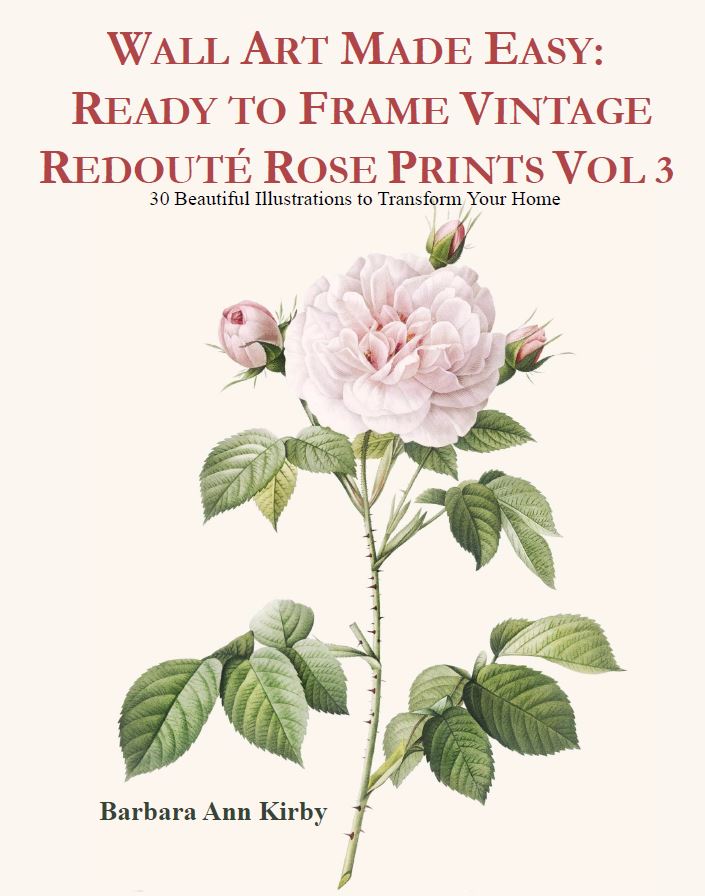The image is the cover of a book titled "Wall Art Made Easy: Ready to Frame Vintage Redouté Rose Prints Volume 3" by Barbara Ann Kirby. The subtitle, "30 Beautiful Illustrations to Transform Your Home," is displayed beneath the title. The book cover features a large, detailed vintage illustration of a pink rose with a darker pink center, surrounded by dark green leaves and several unopened buds. The stem of the rose is light green with visible veins and distinct thorns. The background of the cover is a light off-white color, giving the artwork a classic and elegant look. The title is prominently printed in bold red text, and the author's name is located in black text at the bottom left corner of the cover. This image gives a clear impression of the beautiful, ready-to-frame botanical prints contained within the book.